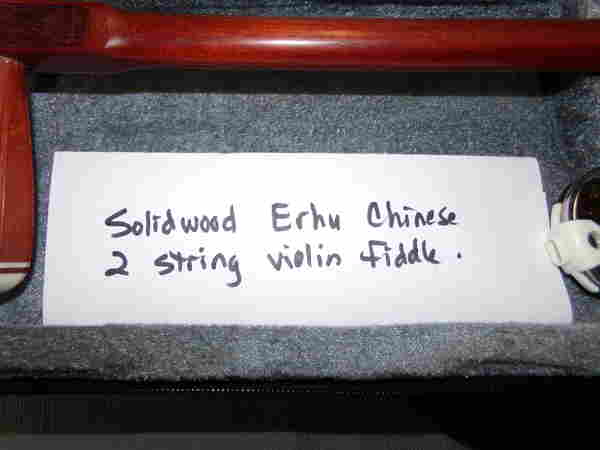In the image, a handwritten sign made from a rectangular piece of white paper lies on top of gray carpeting. The sign reads "Solid Wood Erhu Chinese Two-String Violin Fiddle" in black ink, spread across two lines. The setting suggests a sales advertisement, potentially for an online marketplace. To the right of the sign, a white object that resembles a kettle can be seen. Above and to the left of the sign, there is the partially visible neck and handle of the referenced Erhu, showcasing its reddish-brown polished wood and white trim at the base. The interior of the violin case or another black object is barely visible below the carpeting, adding depth to the scene. The dominant colors in the image include gray, white, black, brown, and silver.